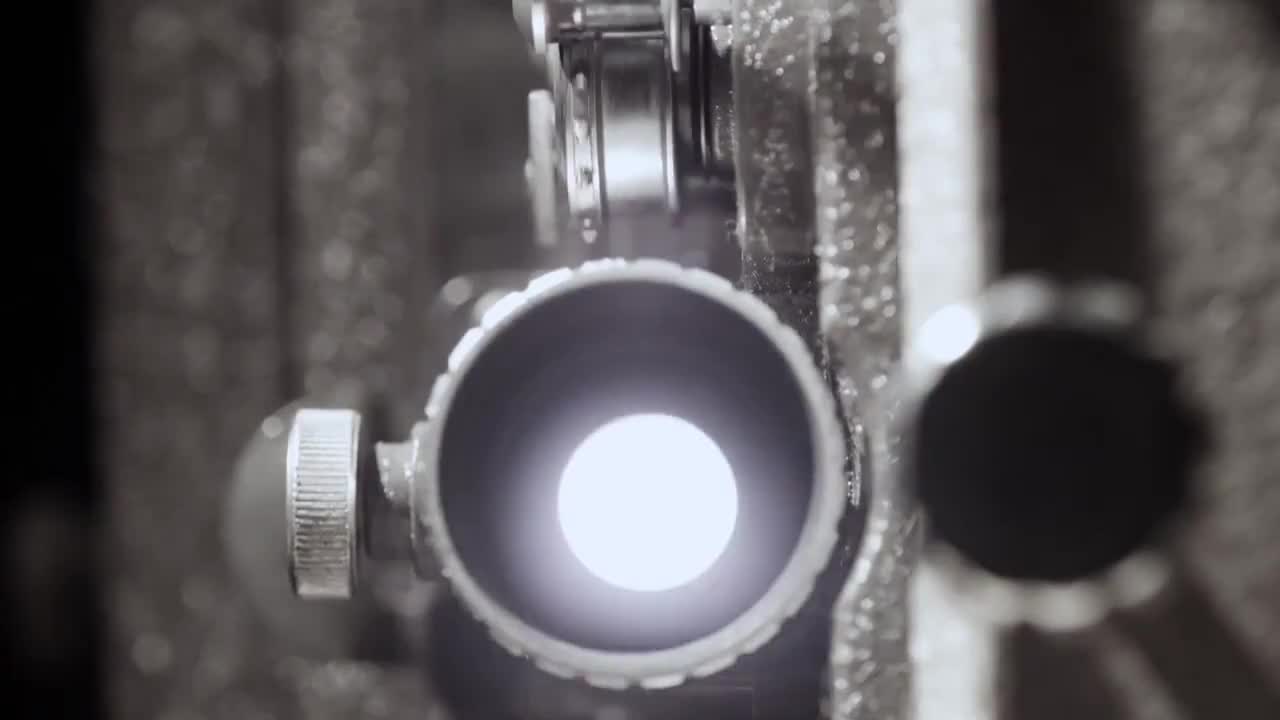The image depicts a detailed close-up of a projector lens, prominently centered and in the process of projecting light, as evident from the light radiating from the lens. The lens has a dark gray body with a textured, ridged surface and a light metallic luster. A tightening dial, located on the side, is visible but slightly out of focus. Above and behind the lens, metallic gears can be seen, contributing to the mechanical complexity of the device. The image has a narrow depth of field, sharply focusing on the projector lens and the gears while rendering other elements, such as a large black knob to the right, slightly blurred. The overall composition highlights the intricate details and textures of the projector lens, set against a monochromatic metallic background.